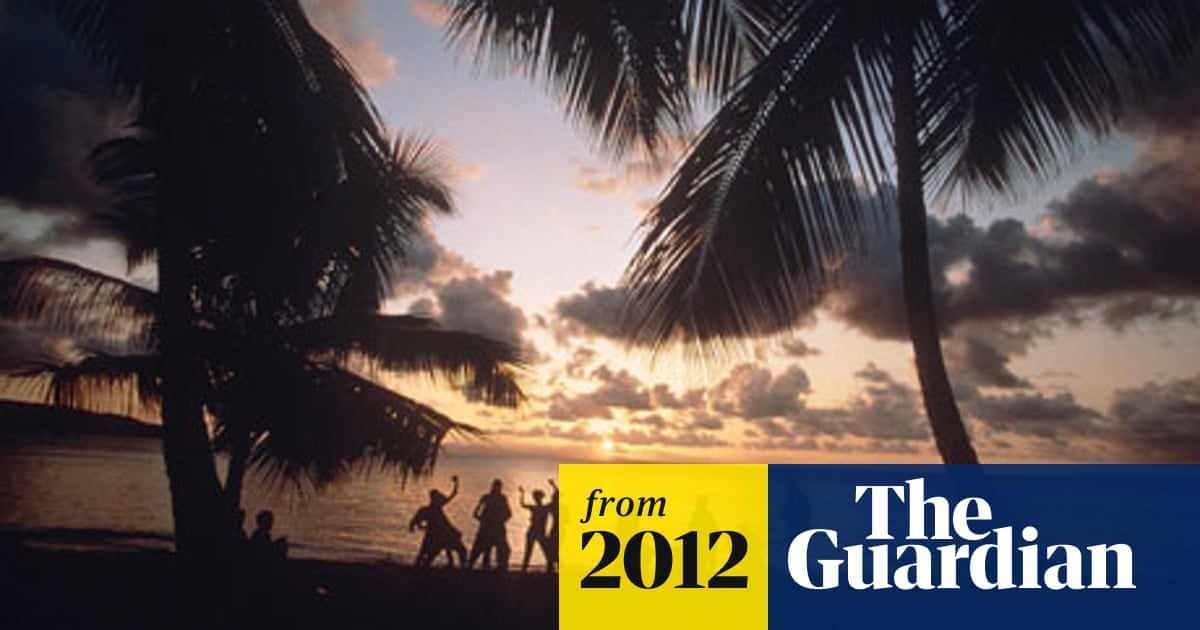This landscape rectangular image, approximately twice as wide as it is high, captures a serene beach at sunset. Dominating the composition are two tall palm trees, one on the left and one on the right, with long, thin leaves and extended trunks. The beach scene reveals three to four silhouetted figures standing near the shore, raising their arms as if in celebration, gazing out toward the setting sun that lies centrally, just above the horizon. The lower portion of the image, especially the bottom right corner, is marked by distinct labeling: a large blue rectangle displaying "The Guardian" in white text, covering at least half of the image's width, juxtaposed with a smaller yellow rectangle bearing "From 2012" in black text. The background showcases a darkening sky with clouds tinged by the twilight hues, and the sea glistens under the sun's fading light, evoking the tranquil beauty of a Caribbean beachscape captured by The Guardian in 2012.